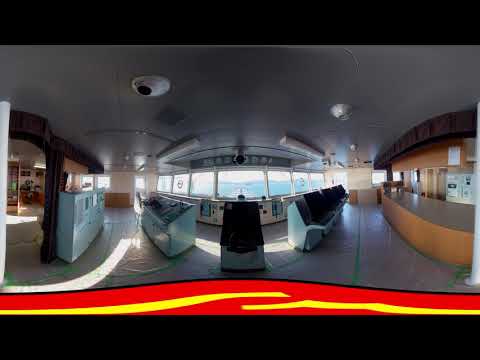The photograph captures the interior of what appears to be the bridge of a ship, possibly a control center on a large vessel. The room is vacant and the atmosphere is slightly dark with natural light filtering through the windows, reflecting on the hard floor and casting shadows. Through the windows, a blue body of water is visible, suggesting the ship is either on a journey or docked. 

In the foreground, there is a digital addition to the photograph—black wavy lines with a bright red and yellow arch just above the letterbox effect at the bottom. Light blue panels equipped with buttons and touchscreens dominate the central area, likely control equipment for the ship's operations. To the left, there are more blue rectangular panels or cabinets, as well as a brown pillar extending to the gray ceiling. The ceiling itself houses several white surveillance cameras. On the right, a brown wall area with two doorways and a countertop, possibly a business desk or support station, is visible. A row of seats is also installed on the right, suggesting a place for crew members or passengers.